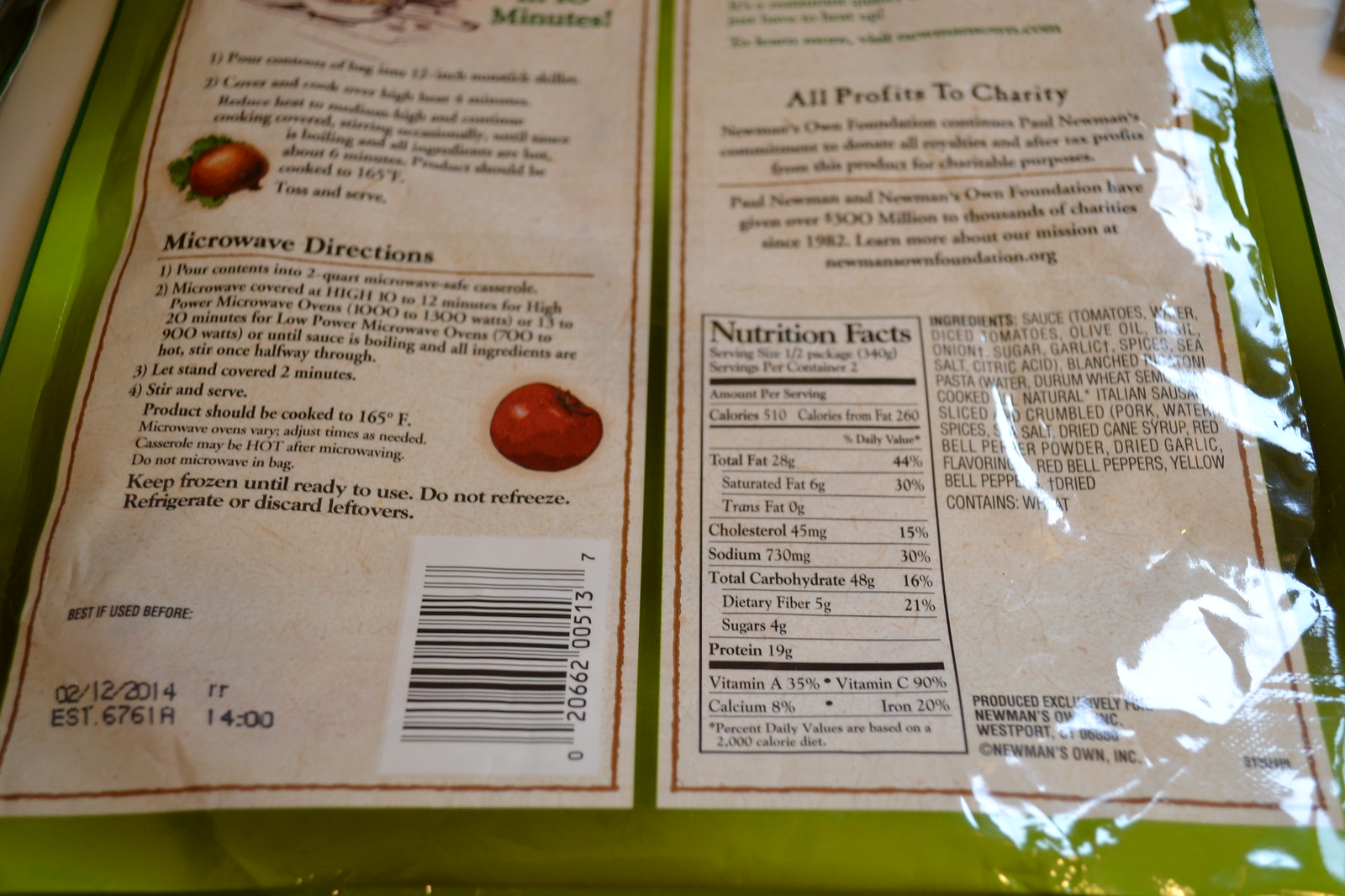The image displays the back of a food package featuring detailed nutritional information. On the left side of the label, there are microwave instructions for proper heating, situated above a notice stating "Best if used before 2-12-2014". Adjacent to this, on the right side, a prominent message reads "All Profits to Charity". Below this declaration, there's an ingredient list that begins with "sauce, tomatoes, water"; however, some details are obscured by a reflection, making the full list difficult to discern. Next to the ingredients, a familiar nutritional facts rectangle provides a comprehensive breakdown of the product's content. This includes measurements for fat, cholesterol, sodium, carbohydrates, and protein. Towards the bottom of this section, the amounts of vitamins A and C, as well as calcium and iron, are also listed.